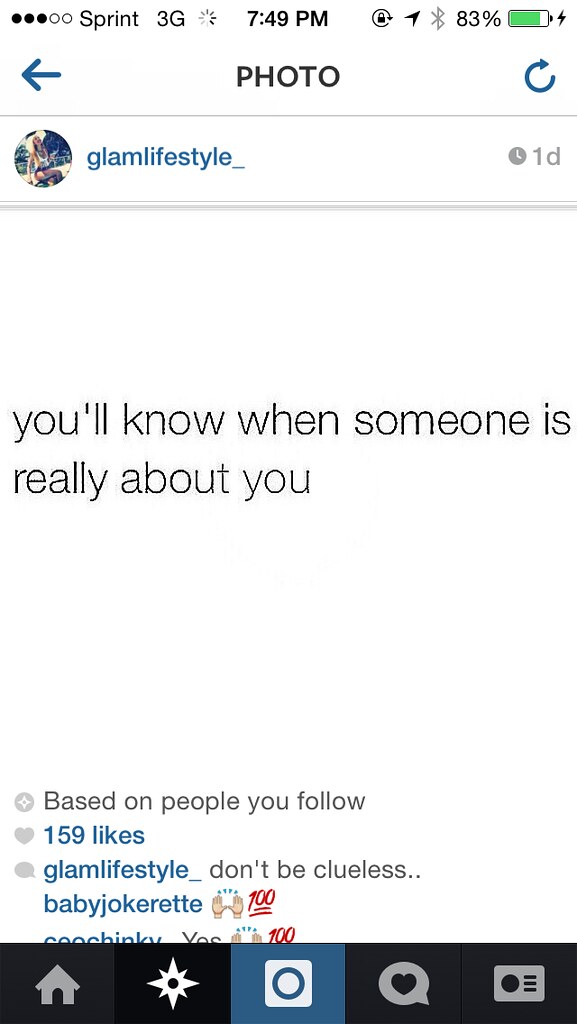This screenshot from a Sprint 3G phone at 7:49 PM with 83% battery displays an Instagram post. At the top, a back arrow is visible next to the "Photo" label. The main image features a photo of a girl from the profile 'glamlifestyle_,' who appears to lead a glamorous lifestyle. Posted one day ago, the image contains a white background with blue and black text. The central message in black reads, "You'll know when someone is really about you." Below it, in blue text, it states, "Based on people you follow," followed by "159 likes." The caption from 'glamlifestyle_' further emphasizes, "don't be clueless... baby joke," accompanied by a hands-up and 100 emoji. The bottom navigation bar on the phone displays icons for Home, Explore, Camera, Notifications, and Profile on a black background.